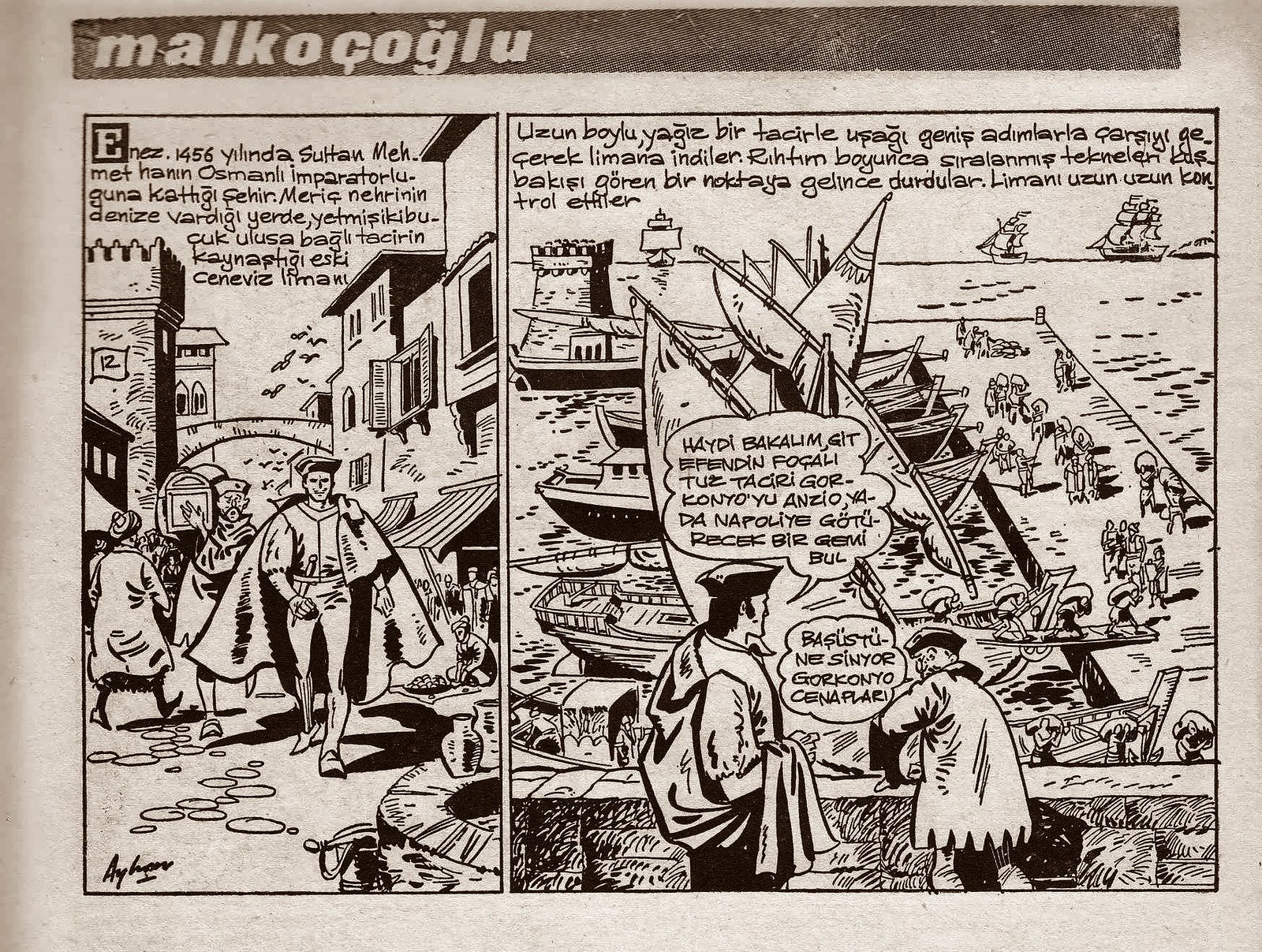This black-and-white comic strip, labeled "Malkoğlu" in bold white letters on a black rectangle at the top, features two detailed panels illustrating a scene from what appears to be a Renaissance or medieval European setting. The first panel, taking up about one-third of the strip, depicts a bustling cobblestone street lined with shops and people. A man with a long, flowing cape, a hat, and a sword tucked into a sheath walks down this street toward the viewer. Trailing behind him is his attendant, struggling under the weight of a large treasure chest slung over his shoulder. Additional details include a well with vases on it in the corner of this panel.

The right panel, significantly larger, shifts the scene to a port with numerous masted ships moored by a dock and a few vessels further out on the water. Here, the caped man stands in the foreground, conversing with a sailor who leans over a stone wall. Speech bubbles and text, all in an unidentified non-English language, are present above both frames and indicate dialogue between the characters.